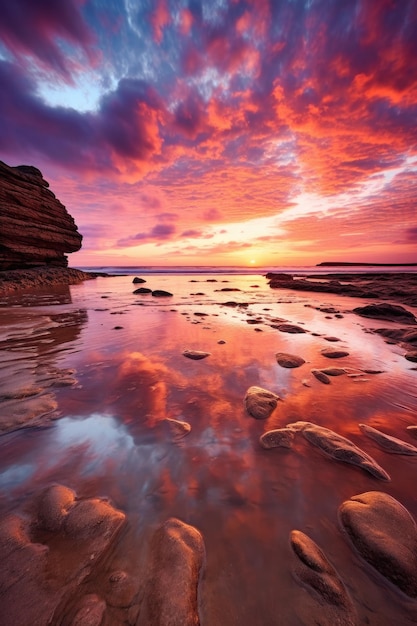This captivating photograph, possibly edited for added vibrancy, captures the serene beauty of a sunset or sunrise over a shallow beach pool. The sky is awash with a mesmerizing palette of pinks, oranges, purples, blues, and light yellows, resembling cotton candy, with the sun nestled amidst fluffy, dense clouds peeking through cracks. The tranquility of the scene is mirrored flawlessly on the calm water below, creating a near-perfect reflection that enhances the dreamlike quality of the image.

The shoreline is punctuated by several rock formations; a prominent, layered outcrop stands majestically on the left, shaped by weathering and erosion, while smaller rocks emerge intermittently from the water and are scattered throughout the middle and to the right. The water’s surface remains mostly undisturbed, with only slight ripples to break its glass-like appearance, adding to the sense of peacefulness and calm.

In the foreground, patches of wet sand are visible, their mounds subtly poking through the shallow water, as if stepping on them would leave a temporary mark. This enchanting scene, with its vibrant reflections and detailed landscape, evokes a sense of pristine natural beauty and tranquil solitude at the edge of an expansive ocean.